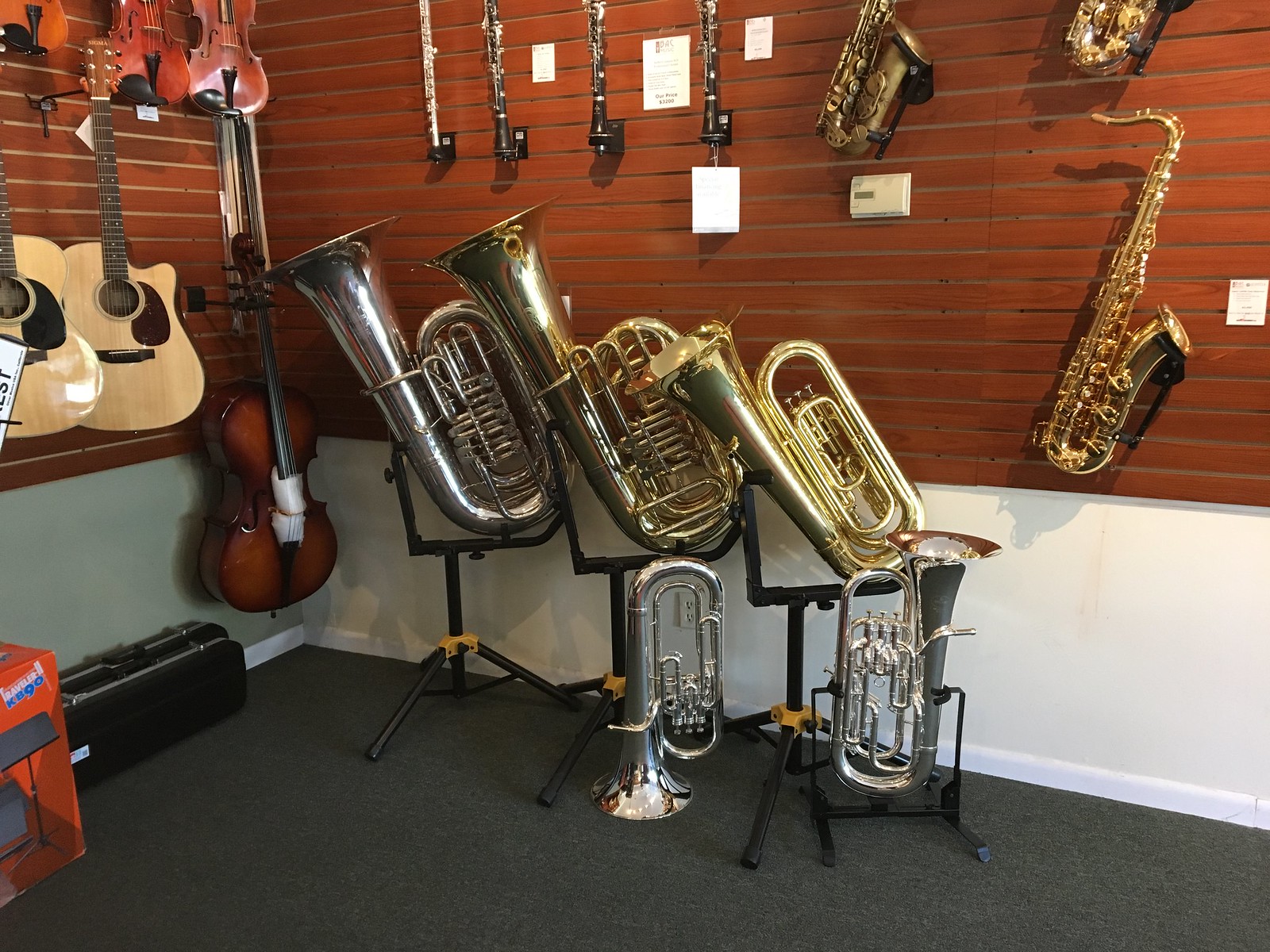The image depicts the inside of a music store, showcasing a rich and vibrant panorama of musical instruments. The scene is set against walls partially clad in cherry wood-colored planks along the upper part, transitioning to white towards the bottom, all resting on a dark gray carpeted floor. 

Predominantly observed in the center are three tubas; a silver one positioned on the left and two golden ones on the right, all supported by black three-legged stands. Around these tubas, a symphony of other instruments catches the eye: smaller silver tubas or perhaps French horns lie closer to the ground. The back wall, robustly adorned with a collection of hanging instruments, displays a variety of saxophones on the right side, flutes above the tubas, and a mix of clarinets.

Moving leftward on the wall, the string section emerges with an array of violins and guitars. Additional details punctuate the scene—a black case and an orange box on the floor contribute to the organized array of musical equipment. The overall ambiance is enriched by the harmonious arrangement of instruments, neatly displayed for what appears to be an inviting and visually appealing musical haven.